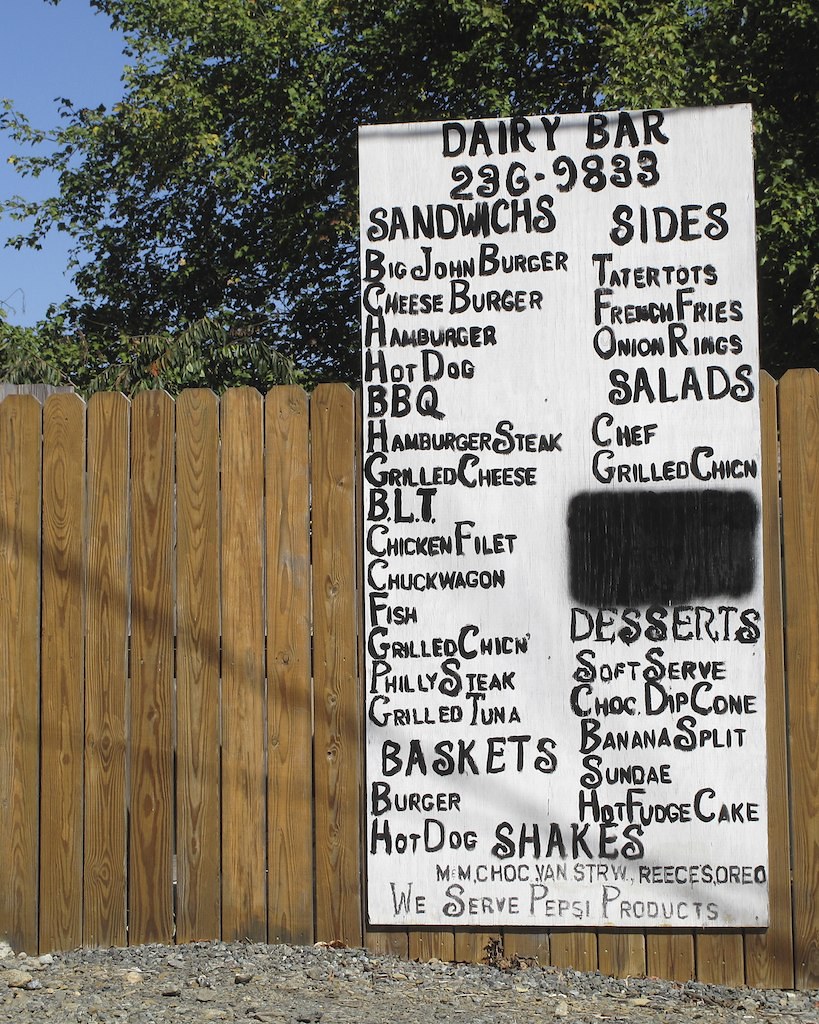The image depicts a light gray wooden fence adorned with a large, hand-painted wooden menu. The menu, painted white with black text, prominently displays "Dairy Bar" at the top, followed by a phone number, 236-9833. The menu is divided into two sections: "Sandwiches" on the left and "Sides" on the right.

The "Sandwiches" column offers a variety of options, listed as follows:
- Big John Burger
- Cheeseburger
- Hamburger
- Hot Dog
- Barbecue
- Hamburger Steak
- Grilled Cheese
- BLT
- Chicken Filet
- Chuck Wagon
- Fish
- Grilled Chicken
- Philly Steak
- Grilled Tuna

Below the sandwich options, there's a "Baskets" category with:
- Burger
- Hot Dog

The "Sides" column lists:
- Tater Tots
- French Fries
- Onion Rings
- Salads (Chef and Grilled Chicken varieties)

A large, black spray-painted square obscures some text in this column. Beneath this, the "Desserts" section includes:
- Soft Serve
- Choc Dip Cone
- Banana Split
- Sundae
- Hot Fudge Cake

At the bottom center, the menu features the "Shakes" section with the following flavors:
- M&M
- Choc
- Van
- Straw
- Reese's
- Oreo

Additionally, it notes that they serve Pepsi products.

The scene is set against a light gray fence casting two dull shadows that resemble branches. The ground is covered with concrete rocks. In the background, behind the fence, a treetop filled with leaves is visible against a blue sky, indicating that the photo was taken during daytime. The image is photorealistic and captures the ambiance of a quaint, outdoor eatery.